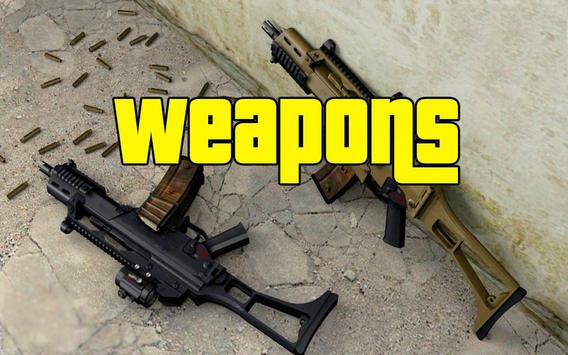This detailed photograph, taken outdoors during the daytime, showcases two automatic weapons positioned on a concrete floor, leaning against a light pale concrete wall. To the right, a brownish-red assault rifle with a large clip and a small handle rests against the wall. This rifle features a thick stock designed for stability. Adjacent to it on the left is a black automatic weapon with a brownish clip and an attached scope. Both weapons are short-barreled and situated diagonally within the frame. Scattered in front of them are numerous bullet casings, suggesting recent use. The image is rectangular, approximately four inches wide and three inches tall, and prominently features the word "weapons" in bold yellow print with a thin black outline at the top center.